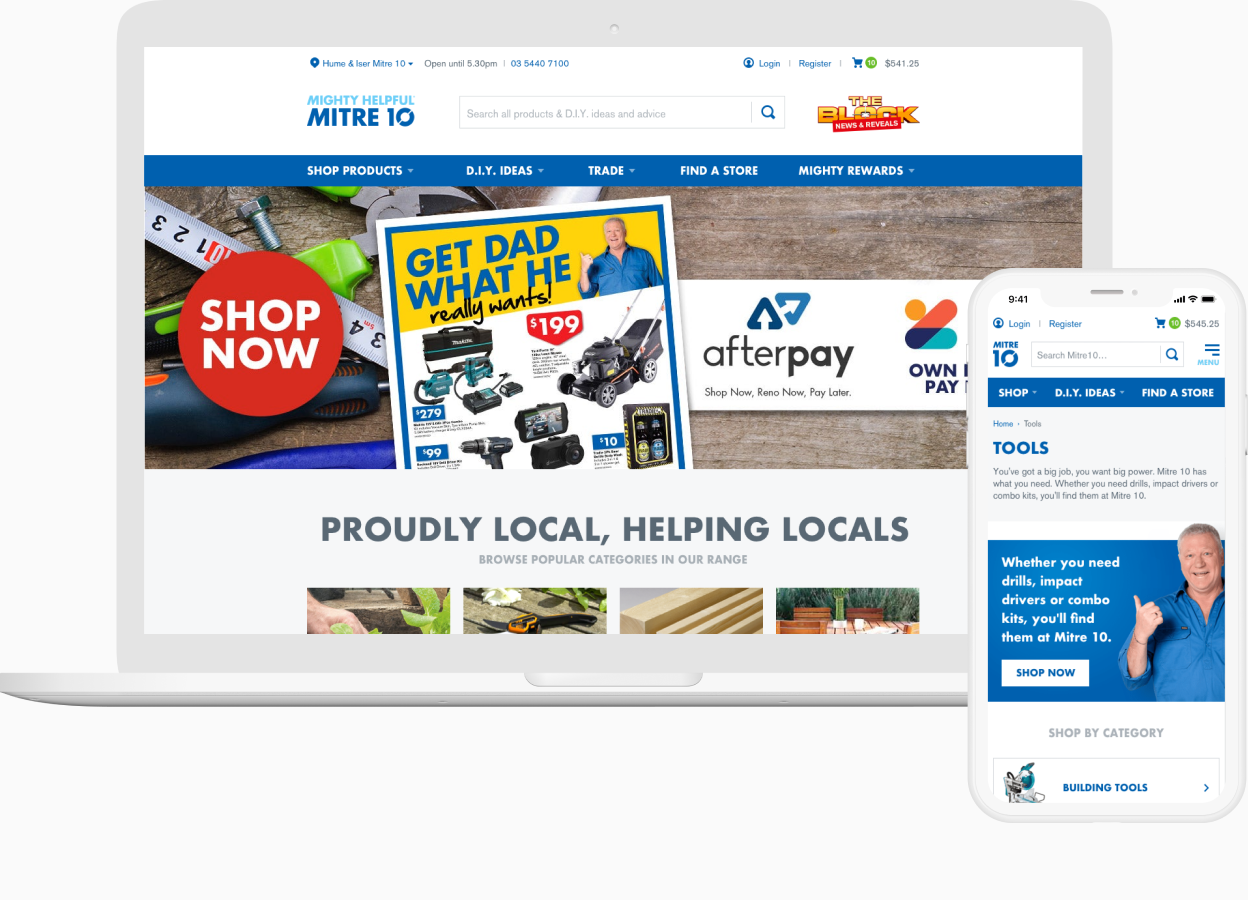The image features a white rectangular computer monitor displaying the Mighty Helpful Mitre 10 website. The background of the image is primarily white. On the right-hand side of the screen, there is a yellow block of text labeled "News and Reveals." In the upper right corner, options for "Login" and "Register" are visible, alongside a blue shopping cart icon indicating there are 10 items totaling $541.25 in the cart.

Centrally located, there is an advertisement showing a man wearing a blue work shirt. The ad encourages viewers to "Get dad what he really wants," featuring options like a lawnmower, a toolbox, and various tools such as a drill and an air compressor. Beneath this, the text reads, "Proudly Local, Helping Locals," followed by an invitation to "Browse Popular Categories in Our Range."